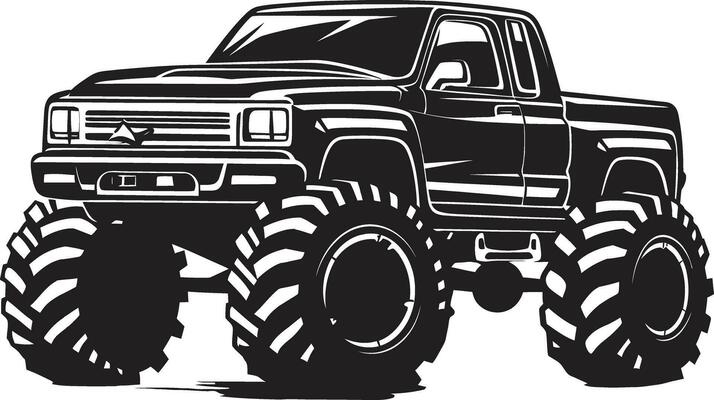A black and white animated image of a lifted monster truck, depicted in a simple and flat art style with no border and a white background. The truck's body is predominantly black, featuring white lines to highlight details such as the grooves on the hood and the outlines of the windows, which are black with white tints. The large, elevated tires are black with white-shaded treads and white-bordered rims, suggesting the need for a ladder to climb into the vehicle. The truck appears to have a short bed and a potential back seat, although the absence of an external handle hints that the back door might open from the inside. The front left tire is notably highlighted with black shading.